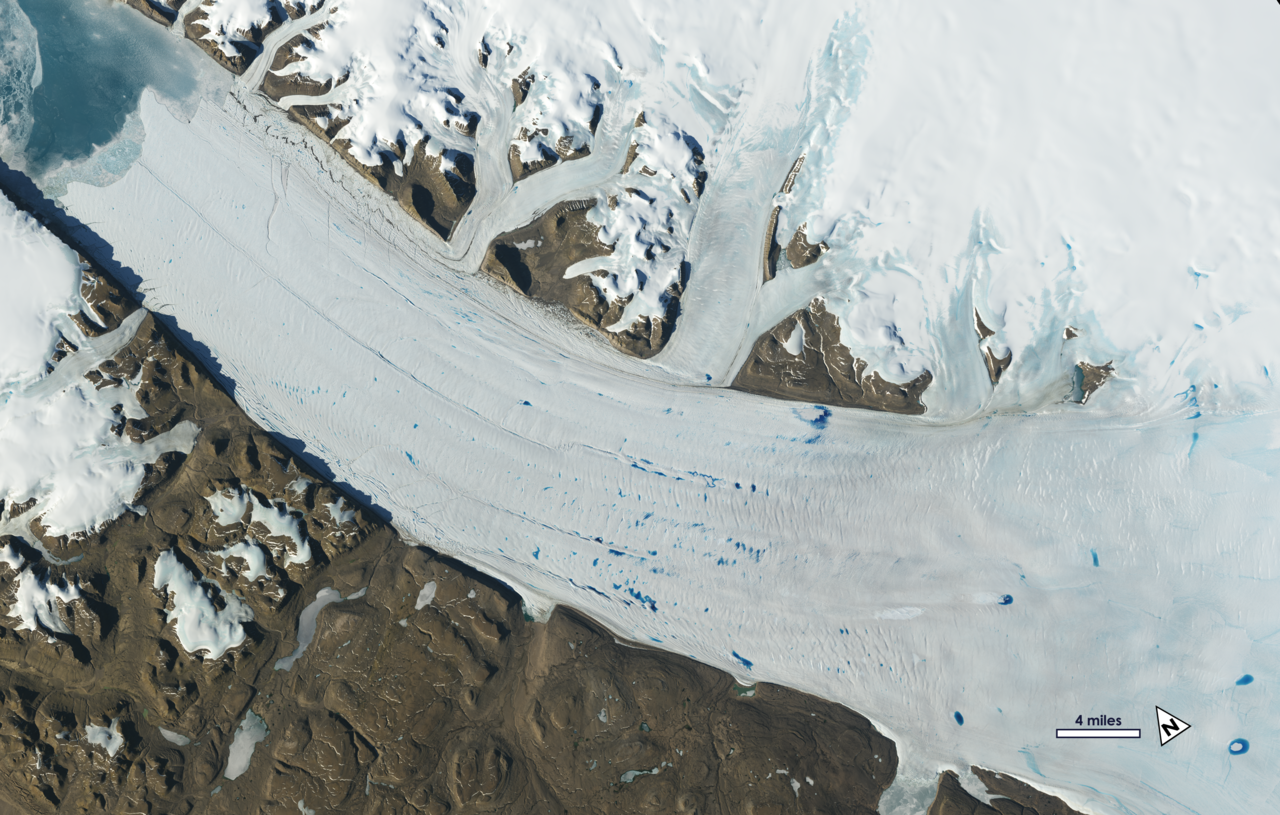This aerial photograph captures a stunning wintry landscape, potentially of a glacier or a river enveloped in snow and ice. From a top-down view, the scene presents a confluence of natural elements that resemble a meticulously detailed painting. In the top left corner, there's a glimpse of ice-cold, blue water, possibly part of an ocean, river, or meltwater from the glacier. This water is largely bordered by a defined pathway that stretches horizontally across the image, accentuated by connected rock formations. 

These rocks are sporadically dusted with snow, more heavily on the right side, where the scene transitions from rocky terrain to predominantly snow-covered and icy expanses. The landscape bears the texture and colors of mountainous regions, appearing as a mix of gray and brownish-gray clay. In the top sections and scattered throughout, there are bright white patches of snow sitting atop elevated areas, giving the impression of capped mountains. The entire composition lends itself to the natural beauty of winter, where frozen rivers, snowy pathways, and rocky mountains converge in a captivating, almost painterly vista.